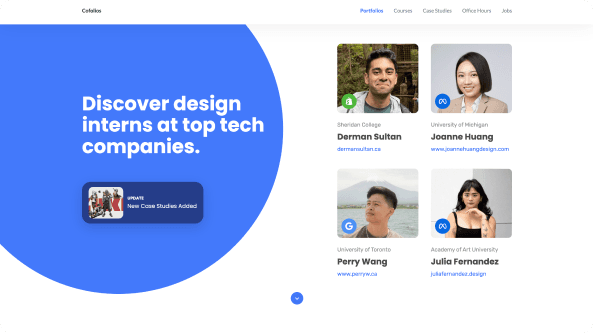On this webpage for a company, a significant portion of the text is too small and blurry to be readable. The design consists of a white background with a prominent bright blue circle located in the upper left quadrant. Inside the blue circle, bold white text reads: "Discover Design Interns at Top Tech Companies." 

Beneath this heading, there is a navy blue button with an inscription in white text that says: "Update." Below the button, smaller white text announces: "New case studies added."

Adjacent to this button, within a white square, there is an image of people, although it is too small to discern their activities clearly. 

To the right of the page, against the white background, four individuals are prominently featured, each with a headshot. Two of them are smiling, one is looking straight ahead without a smile, and the fourth person is gazing off to the side. 

The individuals are identified as follows:
1. German Sultan from Sheridan College
2. Joanne Huang from the University of Michigan
3. Harry Wang from the University of Toronto
4. Julia Fernandez from the Academy of Art University.